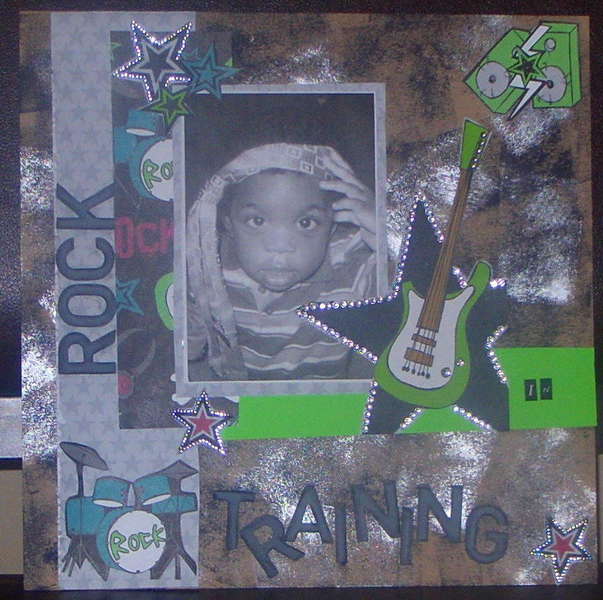The image is a photograph of a homemade, music-themed collage with a graffiti-like style. The centerpiece is a black-and-white photograph of a young Black child wearing a striped shirt and a bandana, reminiscent of Jimi Hendrix. The child gazes directly at the camera. Surrounding the photo is a vibrant mix of objects and colors including pink, green, blue, and white star stickers, glitter, and spray paint in black and white.

On the left side, the word "ROCK" is written vertically in black letters, while at the bottom, the word "TRAINING" is positioned horizontally next to an animated, turquoise drum set with silver cymbals and a white drum head. The drum set has the word "rock" emblazoned in green lettering on the front of the kick drum.

Additionally, the right side of the collage features a green guitar with a white body and a brown neck, and nearby is a large, black star encased with small round jewels. Above the black star, there are two green speakers adorned with a white lightning bolt and a star in the middle. The collage has a dynamic, energetic feel, with letters appearing to dance around the composition, evoking a sense of rhythm and music. The entire piece is set against a brown, charcoal-esque background.